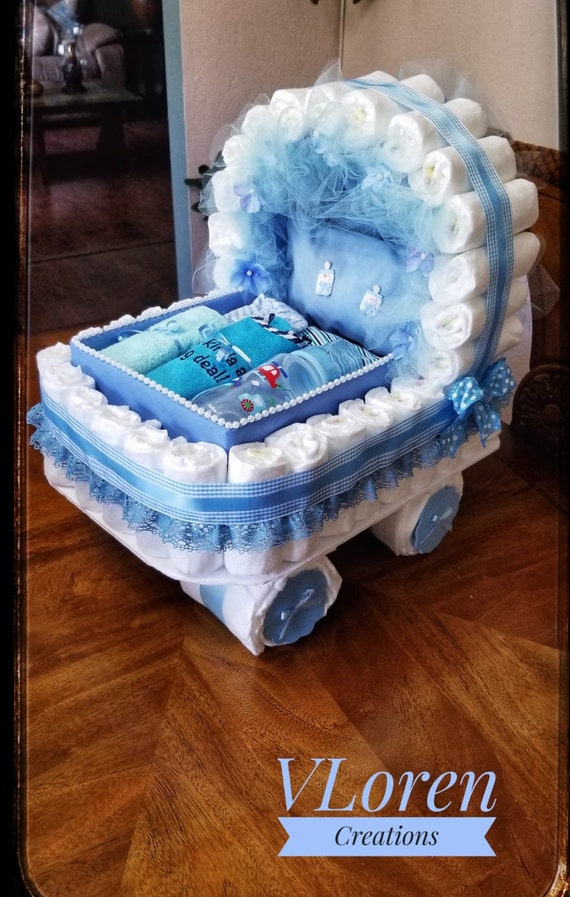This vertical rectangle image features a custom creation from "V. Lauren Creations," as indicated by the light letters and light banner text at the bottom right corner. The main focus is an intricately designed, blue and white baby carriage knick-knack crafted primarily from rolled-up diapers. The diapers form the foundation and the arched back of the carriage, with some creating the wheels wrapped in tissue. Blue and white ribbons, along with lacy blue material, embellish the exterior, and a prominent blue and white bow accentuates the left side where the back meets the side of the carriage. Inside, a blue lining with a white beaded top houses three rolled-up materials in green, blue, and purple. Accompanying the carriage is a small care package containing a baby bottle, baby clothes, and a blanket. All of this is set against a wooden table with a distinct wood grain pattern.